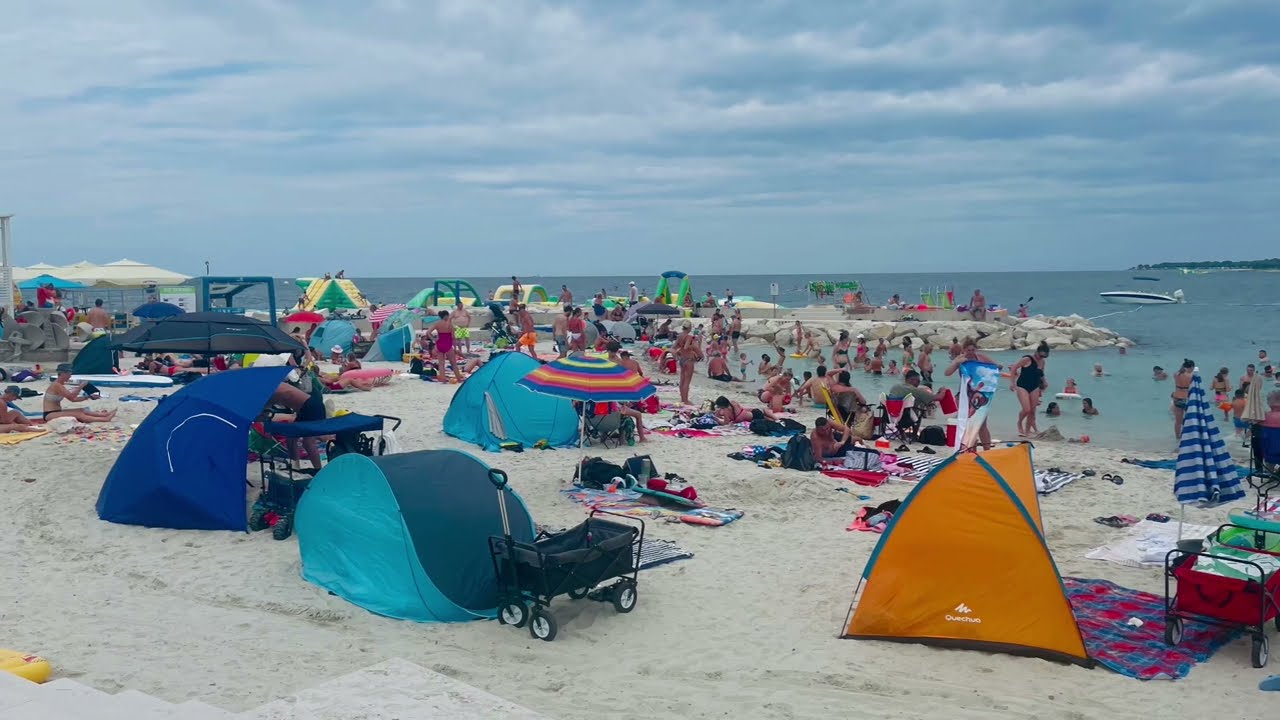This photograph captures a very crowded and bustling beach scene on a cloudy day. The tan sand is almost completely covered with hundreds of people, most of whom appear to be Caucasian, engaging in various activities. The foreground is teeming with a mix of colorful items including tents, beach towels, wagons, and umbrellas. A prominent feature is the array of tents in various shades of blue and orange, such as a two-tone blue tent with a wagon beside it and a larger orange tent on the right-hand side. One particularly vibrant umbrella has a rainbow pattern. The beach is populated by people sitting, lying down, walking, and playing both on the sand and in the shallow waters near the shore, where there's a shoal visible. A small boat is also seen navigating the open water in the background. The far side of the image depicts another shore across the sea or ocean, but much of the focus remains on the lively activities closer to the camera. The sky is marked by large, fluffy clouds, creating an overcast ambiance without being too dark, making it a fun and energetic gathering for beach-goers.